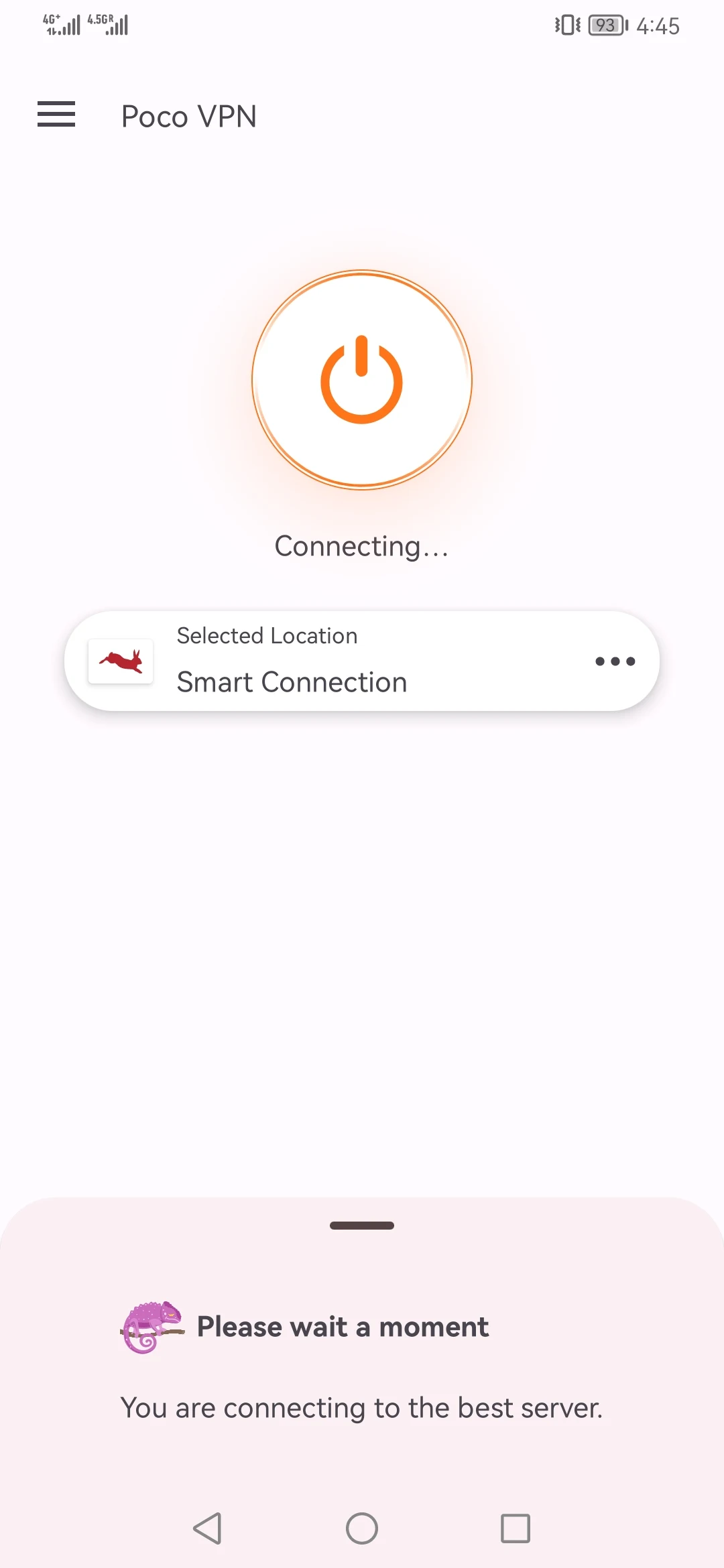The screenshot displays a smartphone interface for a VPN application titled "Poco VPN." The device shows its status in the top left corner: "4G, Vibranium 4," and in the top right, a battery icon reads "93%." The central focus is a large red power button with orange edges, featuring a traditional power symbol (a circle with a line through it). 

Above the power button is a hopping bunny icon, adjacent to which is an oval indicating the "smart connection" feature. The background of the interface is predominantly white, transitioning to pink and purple hues at the bottom. Alongside, a chameleon with a wavy, spiral tail is perched on a branch, adding a touch of whimsy.

Text at the center of the screen reads, "Please wait a moment," followed by "You are connecting to the best server." Additional icons include a sideways triangle, a circle, and a square. The overall aesthetic is playful yet functional, with a screenshot indicative of an in-progress connection setup on the VPN app.